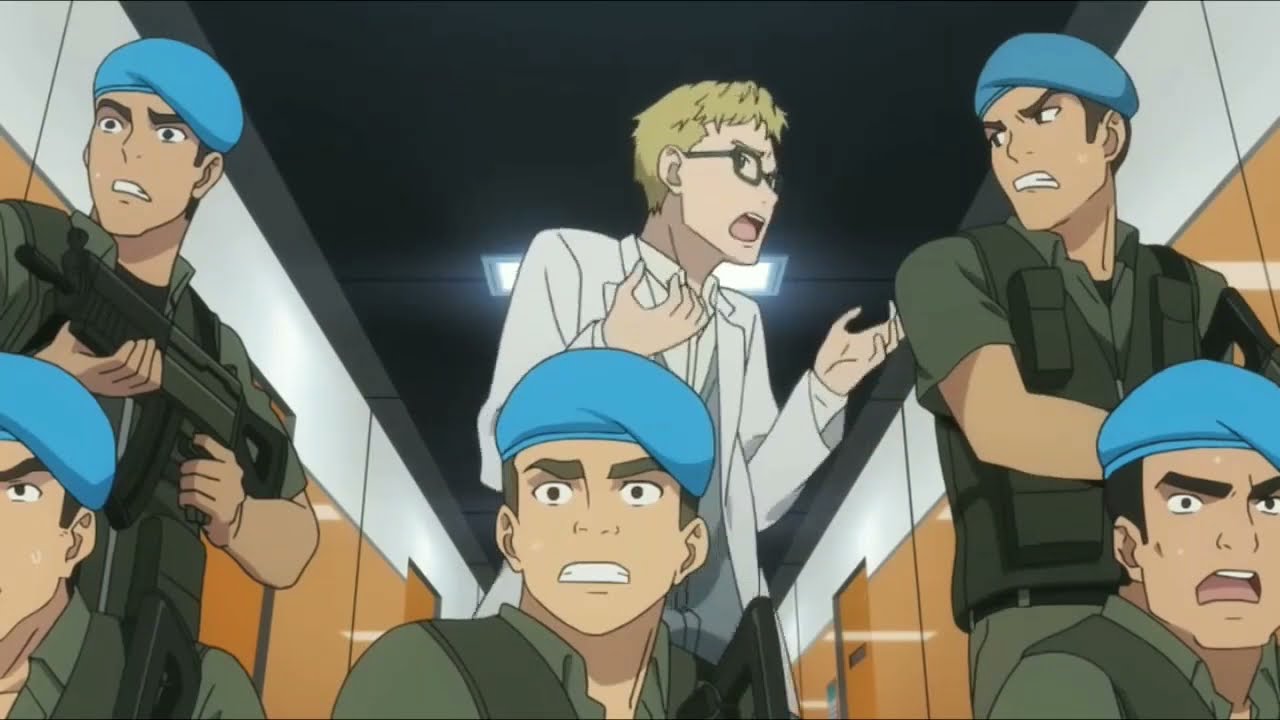This scene, drawn in the style of Japanese anime, depicts a tense moment inside a building hallway with orange walls and white upper sections. The black ceiling features a white rectangular light. There are six men in the image: five soldiers and one individual who appears to be a scientist. The soldiers, all wearing military-green outfits and blue berets, display expressions of fear and intensity with clenched teeth and wide eyes. Two soldiers are positioned on the left, one in the center, and two on the right. Only the upper halves of the men in the foreground are visible, while a soldier on the left, partially obscured, is holding a machine gun. The central figure, the scientist, stands out with his blonde hair, dark glasses, white shirt, gray vest, and white lab coat. His hands are raised to his chest with fingers bent, as if he is pleading or trying to reason with the soldiers. His mouth is open, revealing his tongue and top row of teeth. He is turned towards a soldier on his left, who is looking back at him with a furrowed brow and clenched teeth, seemingly agitated or cross. The atmosphere is charged, indicating a critical confrontation taking place in this hallway.